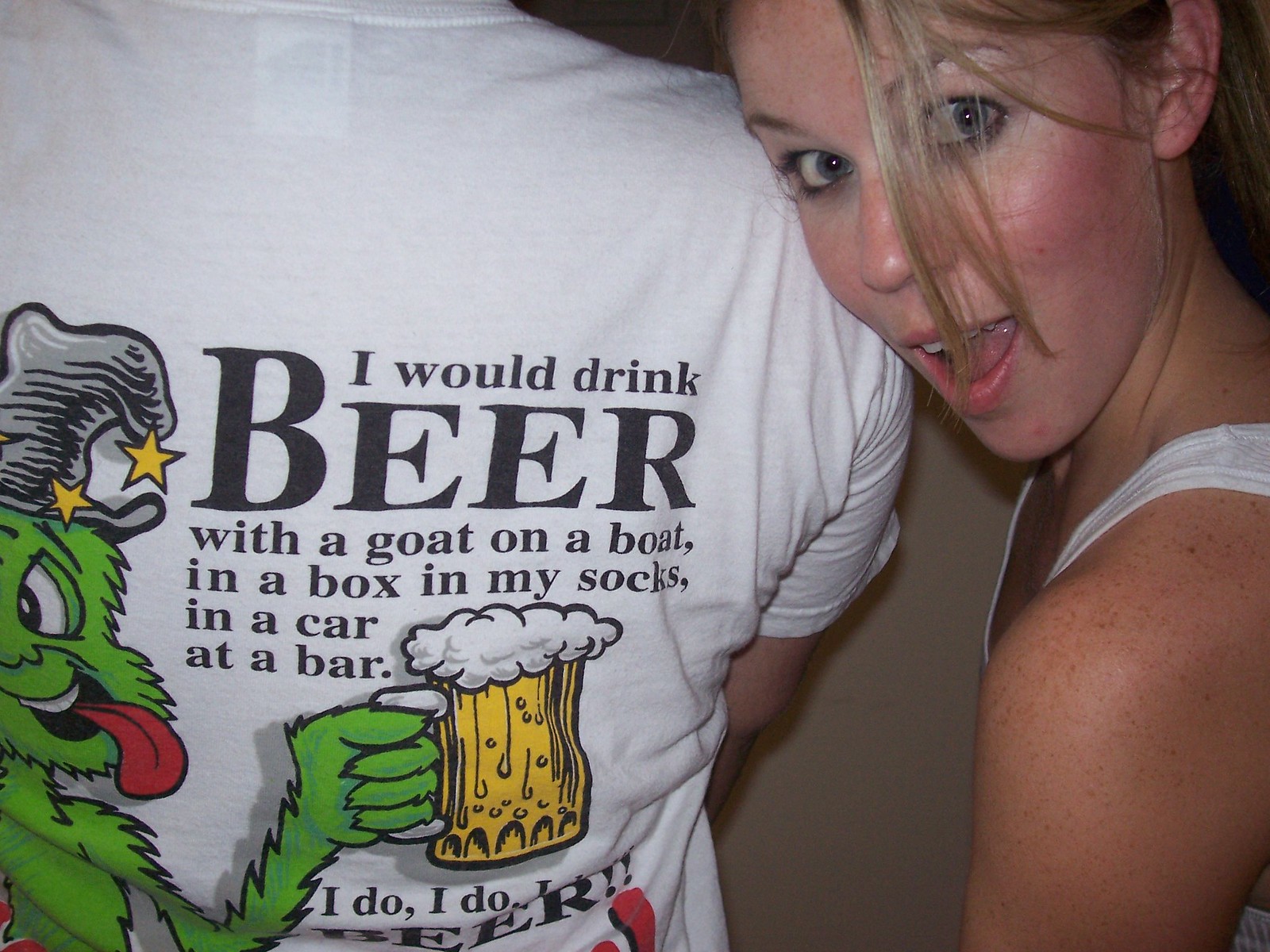In the image, there is a young woman on the right side, leaning her head against the right shoulder of another person whose back is turned to the camera. The woman has blue eyes, pink lipstick, and a white sleeveless top. Her mouth is slightly open as she looks directly at the camera with an excited yet playful expression, her freckled shoulder clearly visible. The person she's leaning on has broad shoulders and is wearing a white t-shirt that has the tag visible through the fabric at the neckline. The back of the t-shirt features an illustration of a whimsical creature resembling the Grinch, with its tongue sticking out and wearing a floppy black hat. The creature is holding a beer mug with foam overflowing, surrounded by stars, and the shirt bears the caption: "I would drink beer with a goat on a boat, in a box in my socks, in a car at a bar. I do, I do, I do, beer." The focal point of the image is the woman's expressive demeanor, contrasting with the humorous and detailed illustration on the man's shirt.